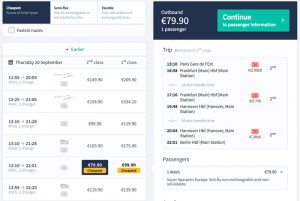The image depicts two highly blurred cell phone screenshots side by side, with a predominantly white background. On the left-hand side, the screen shows a user interface with three selectable options at the top, where the leftmost option is highlighted in navy blue, suggesting it is the active screen. Below that, there are seven visible search results organized into four columns. Notably, the second result from the bottom features two distinct icons. In this particular row, the last two columns contain different elements compared to the rest.

The right-hand screenshot is topped with a solid navy block that displays a price of 79.90 euros. Adjacent to this price block, within the same navy section, is a tea green block containing white text. Beneath this header, there are three visible results, also arranged in four columns. The bottom section of this screen contains additional content, but it is too small to decipher clearly.